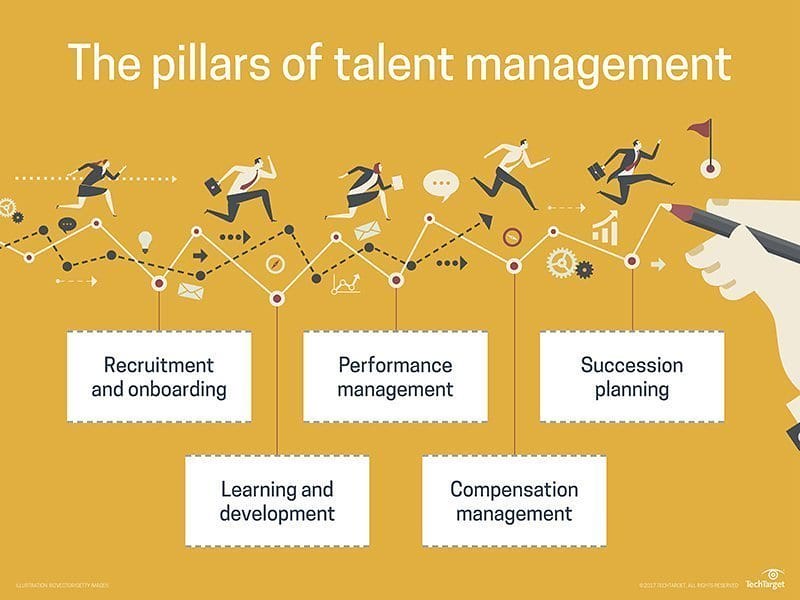This vibrant color image depicts a business infographic set against a marigold yellow background. At the top, white text prominently reads "The Pillars of Talent Management." Below the title, five cartoon characters, dressed in business attire and carrying briefcases, are running along lines of what resembles a bar graph. These lines extend vertically, and the running figures illustrate a dynamic race towards a finish line marked by a flag. The runners consist of three men and two women, all shown in mid-stride. Adjacent to the right side of the image, a cartoon hand holding a pen is actively drawing the lines of the graph. 

Beneath the animated figures, there are five rectangles each containing a key element of talent management. The sections are labeled: "Recruitment and Onboarding," "Performance Management," "Succession Planning," "Learning and Development," and "Compensation Management." The overall effect is a visually engaging representation of the components of effective talent management.